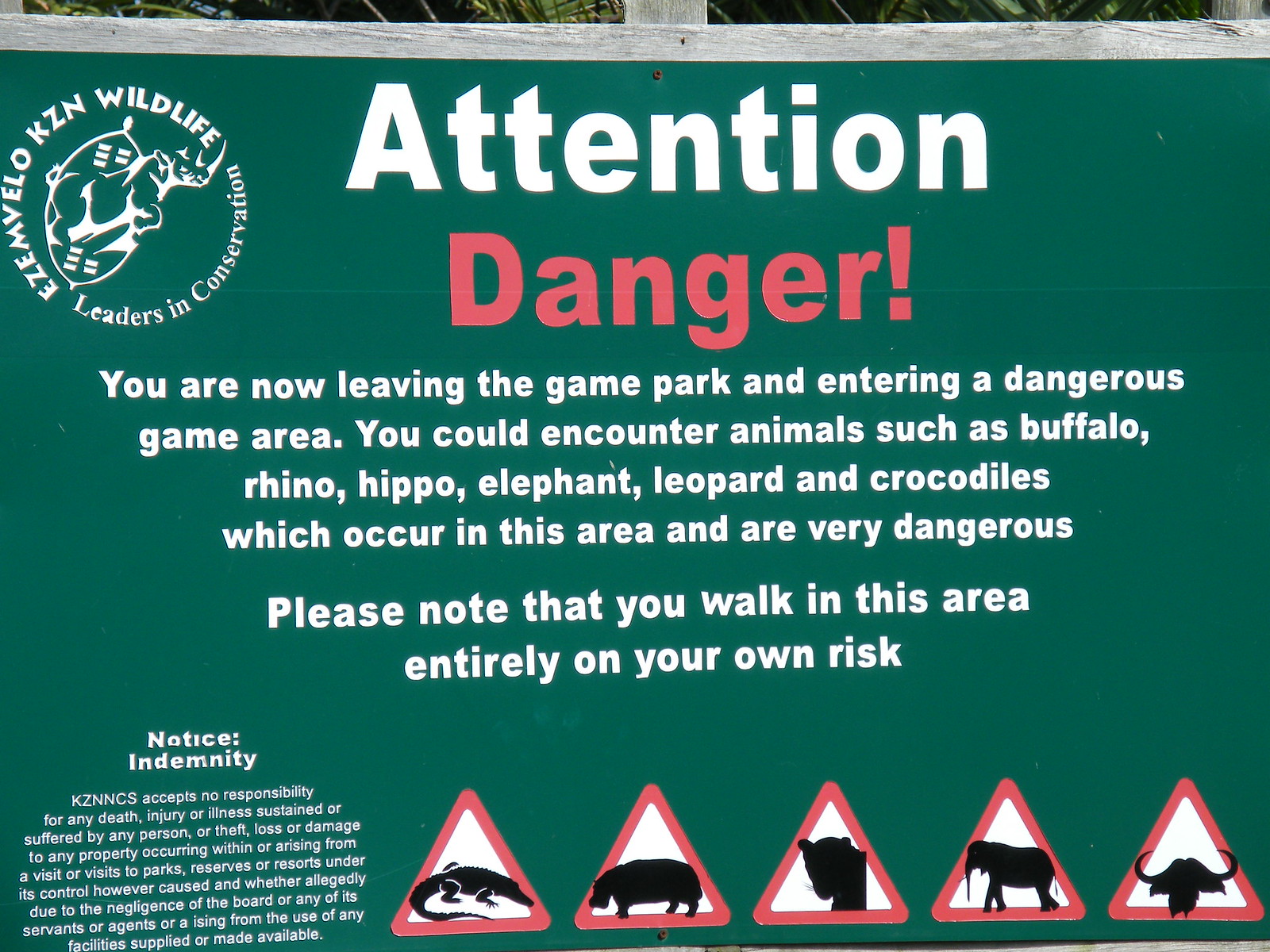The image depicts a large, horizontally oriented, green metal sign attached to a background of light gray wooden boards, indicating an outdoor setting. The sign features prominently white text at the top that reads "ATTENTION," followed by bold red text that says "DANGER!" Directly below, in smaller white text, it warns: "You are now leaving the game park and entering a dangerous game area. You could encounter animals such as buffalo, rhino, hippo, elephant, leopard, and crocodiles which occur in this area and are very dangerous. Please note that you walk in this area entirely at your own risk." At the upper left of the sign is the logo for "Izimailo KZN Wildlife Leaders in Conservation," a round insignia. The lower left corner includes a "Notice Indemnity" with specific legal text about responsibilities. At the bottom of the sign are five red-bordered white triangles, each containing black icons for the animals listed: a crocodile, rhino, hippo, elephant, and buffalo.